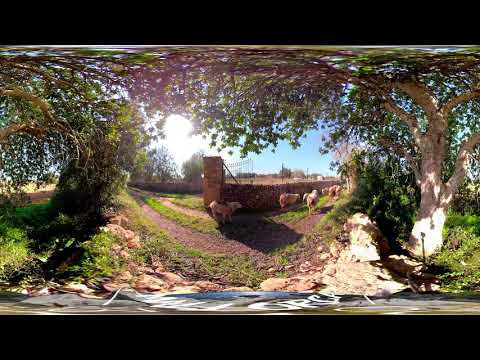This panoramic outdoor photograph captures a serene rural scene through a lens that creates a rounded distortion, giving the image a unique curvature. Central to the composition are two prominent trees with lush green canopies, their strong trunks anchoring the verdant view. Below the trees, a narrow, dark-colored pathway meanders through the landscape, forming a U-shape that suggests it might be part of a driveway. This pathway is surrounded by green grass and occasional rocks, adding to the natural texture. The foreground reveals a strip of camera edge and a thick black border frames the image from the top and bottom.

Behind the trees and paths, a stone or brick wall stretches across the scene, its texture blurred by the soft lighting. Grazing in front of this wall are a number of animals. Initially indistinguishable due to their distance, a closer look reveals white or cream-colored sheep moving away from the viewer, though one shape near the middle could be mistaken for a dog. Further right, additional sheep are visible, creating a soothing pastoral setting. The photograph also captures the sunlight filtering through the trees, casting a gentle glow over the foliage, with the edges of the canopy illuminated against the sky. The mix of natural elements and the subtle play of light evoke a peaceful countryside atmosphere.